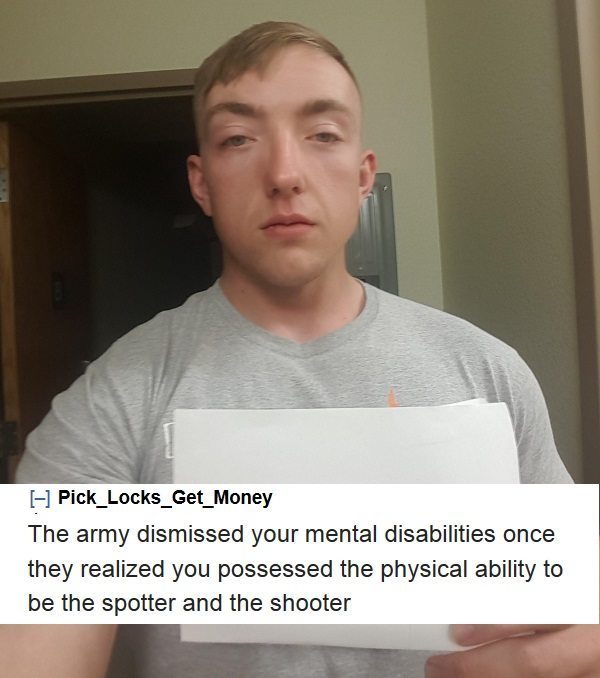This color photograph features a young Caucasian man, centrally positioned in the frame. His short, blondish-brown hair is neatly combed over to the right side. He looks straight ahead, albeit slightly downward, with his mouth downturned, giving him a somewhat sad expression. His notable, disproportionately large cheeks stand out against his otherwise ordinary features, which include moderately open, indistinctly colored eyes and brownish eyebrows.

The man is dressed in a light gray, short-sleeved t-shirt and holds several papers in his left hand, positioned across his torso at the level of his chest and stomach. Notably, the image is overlaid with a white rectangle containing black text at the bottom. The uppercase header reads "PICS_LOCKS_GET_MONEY," followed by three lines of text in a typewriter-style font: "The army dismissed your mental disabilities once they realized you possessed the physical ability to be the spotter and the shooter."

The background reveals an indoor setting with an open doorway on the left and a wall corner on the right. Additional elements like a metal panel on the wall contribute to the contextual surroundings. The combination of visual details and the imposed text suggests a deliberate, possibly humorous captioning of the man's image.